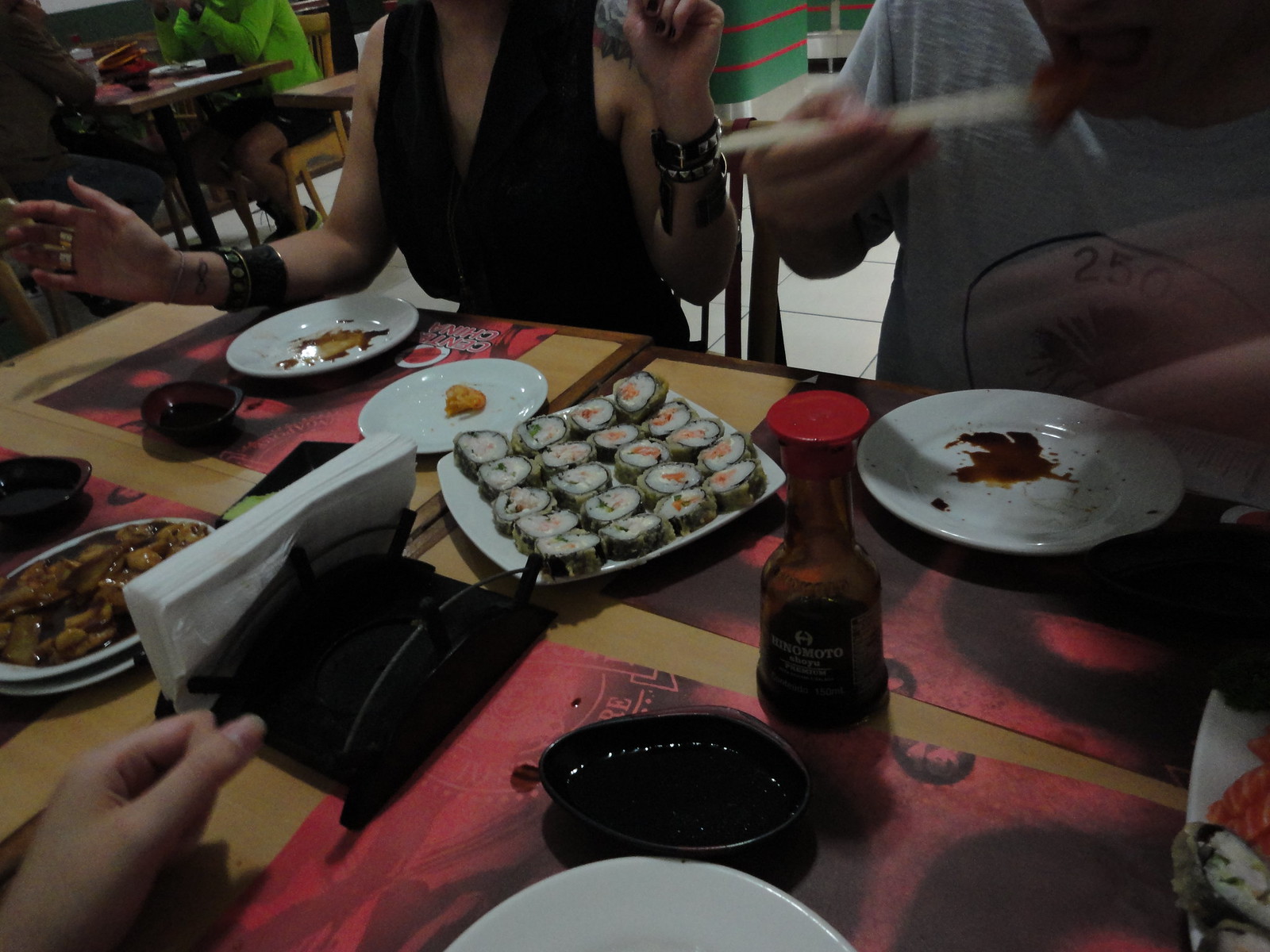This indoor photograph captures a lively scene at a restaurant where five individuals are gathered around a light yellowish wooden table with dark brown edges. The table is adorned with red and black placemats featuring an indiscernible design, and a white plate brimming with sushi rolls sits at the center. Accompanying the sushi is a dark brown bottle of sauce with a red cap. Several other dishes, including a plate of food resembling chicken in sauce, are visible on the table.

In the foreground, a woman in a low-cut black sleeveless dress with black bangles and a tattoo on her left shoulder is sitting. Another lady wearing a light blue shirt and holding chopsticks is lifting a piece of sushi towards her mouth. Near her, a man in a grey t-shirt with the number "250" written on it is also using chopsticks. The hands of two more women, one with longer fingernails, are visible, both interacting with their plates of food.

In the background, a man in a bright green long-sleeve shirt and black shorts is partially visible, further adding to the dynamic atmosphere of the restaurant. Some paper napkins are scattered on the tabletop, highlighting the casual, lively mood as people enjoy their meals and socialize.